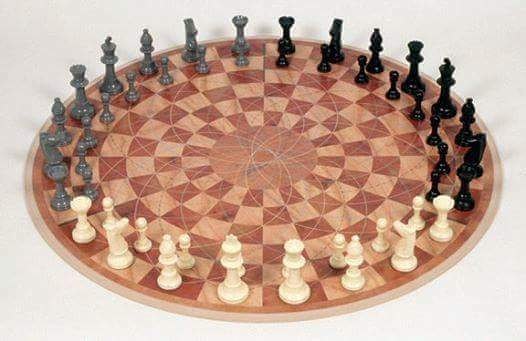This photograph captures a unique, circular chess set, positioned on a pristine white surface, possibly a table or counter. Departing from the traditional square or rectangular board, this one consists of concentric circles with an intricate spiral graph design that extends across all the squares. The color scheme of the board features muted brown and beige checks, overlaid subtly with white spiral lines.

Intriguingly, the chess set accommodates three players rather than the conventional two. On one side, cream-colored chess pieces are lined up in the outermost rows. To the left, gray pieces stand in formation, while black chess pieces are arrayed on the right. The pieces themselves appear to be made of smooth, reflective ceramic, adding a touch of elegance to the set. The photograph is taken from a roughly 70-degree angle, clearly showcasing the unconventional but mesmerizing design of this tri-player chess game.